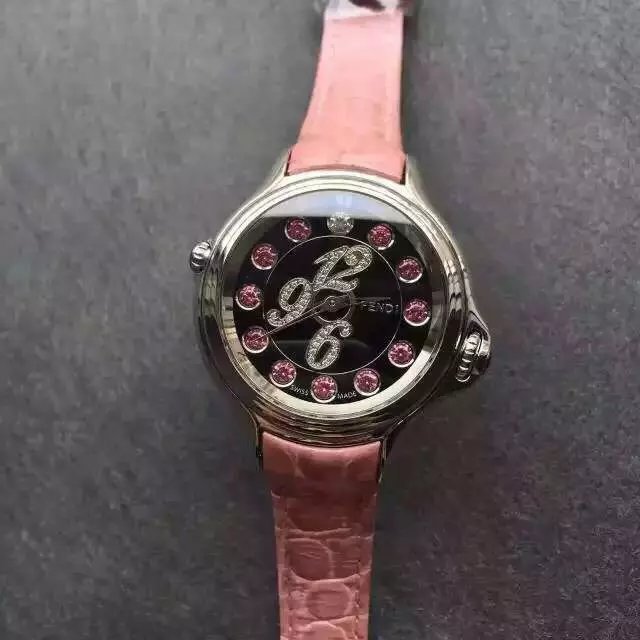This is an intricately detailed photo of a stylish women's watch, taken with a product placement style to showcase its features. The watch is prominently displayed face-up on a textured, light grainy gray background. The band is crafted from pastel baby pink alligator skin leather, giving it a luxurious and feminine touch. The round watch case is silver, and the watch face itself is a deep black adorned with jewel markers for the hours—pink diamonds for most hours, except for a striking white diamond at the 12 o'clock position. Additionally, the inner circle of the watch face features shiny silver numbers at the 12, 9, and 6 o'clock positions. The watch has delicate silver hands, with the minute hand being more prominent. To the right of the watch face, the brand name "Fendi" is inscribed in elegant silver text. The watch also features two knobs, with the larger one positioned on the lower right and a smaller one on the upper left, adding to its functional and aesthetic appeal.